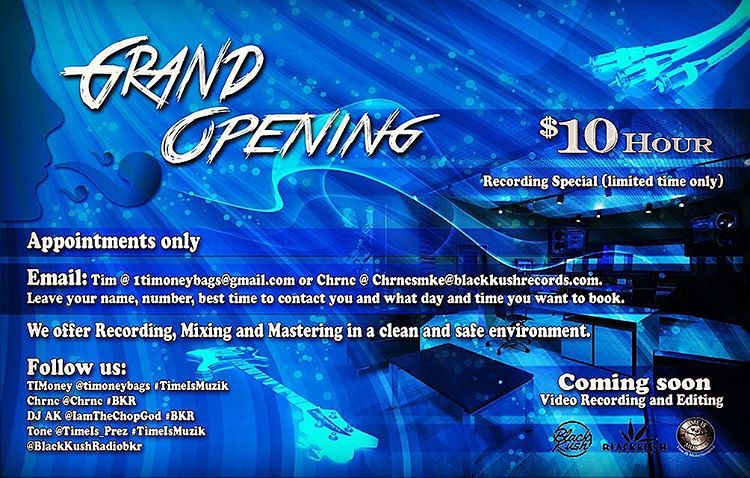This landscape-oriented graphic features a dynamic blue background in various shades, adorned with spacey swirls and lighter blue circles. In the upper left corner, there's a silhouette of a person's face exhaling. The upper right corner includes an image of cables, reminiscent of monster cables. The lower left showcases an electric guitar, while the lower right displays what appear to be boxes—possibly electronic equipment or cabinets. 

White text in the upper right announces "Grand Opening" alongside a limited-time offer: "$10/hour recording special." Below, the graphic states "appointments only," directing inquiries to email Tim at itimoneybags@gmail.com or chrnc at chrncsmke@blackrushrecords.com. It instructs to leave your name, number, best time to contact, and desired booking day. The bottom half emphasizes services like recording, mixing, and mastering provided in a clean, safe environment. The lower left corner includes social media links, and the lower right hints at future services: "coming soon, video recording and editing," accompanied by assorted logos.